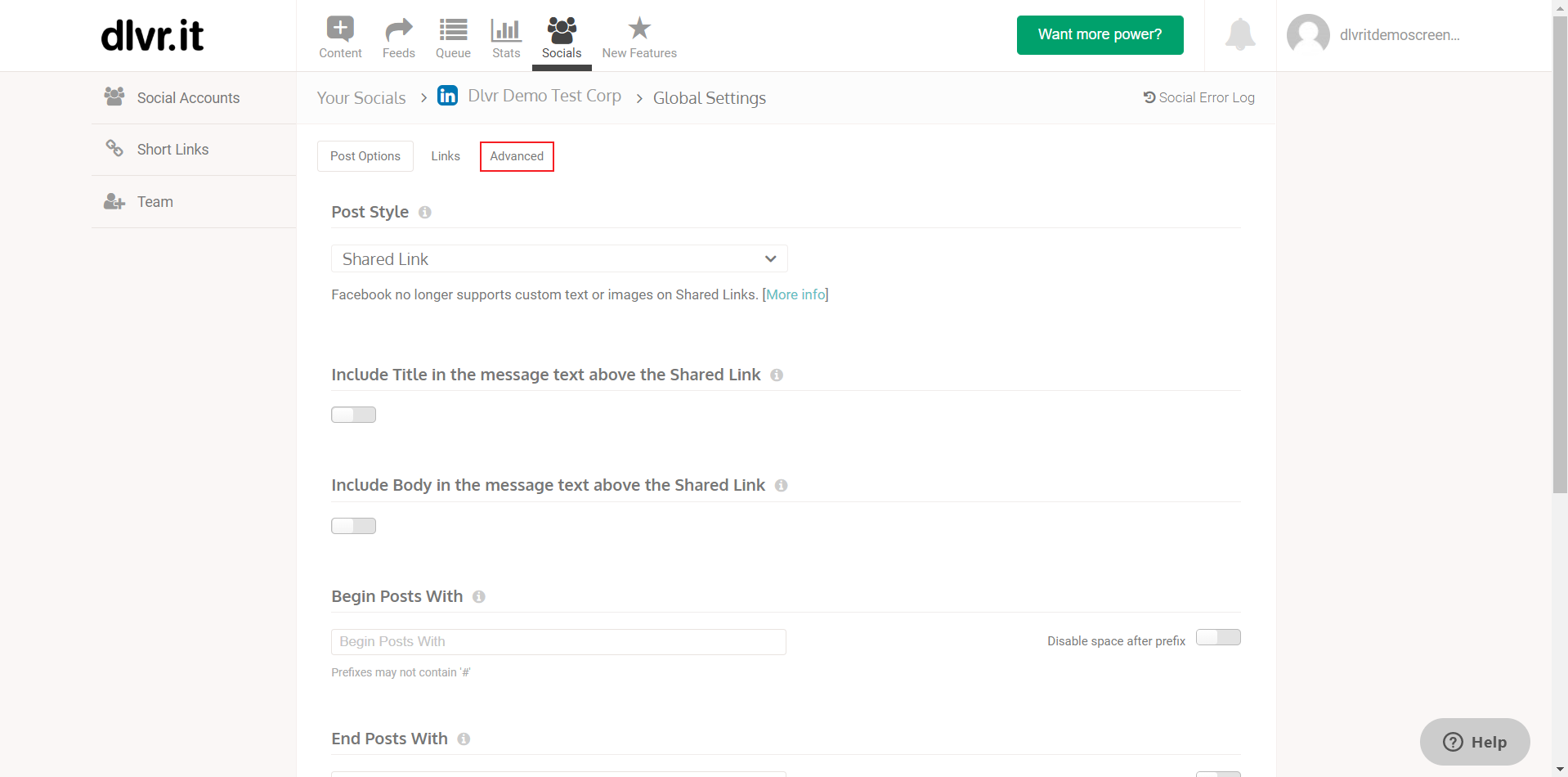In this detailed setting screen of the DeliverIt app, the top left corner features the app's name "deliver.it" in lowercase black letters. Directly below the web page title, three sections—Social Accounts, Short Links, and Team—are listed in gray text on a light gray background, indicating inactive or secondary options. 

On the top right side of the web page, you can find several icons labeled Connect, Foods, Quay, Stats, Schools, and New Features. Adjacent to these icons is a prominent green box with the text "Want More Power?" followed by a light gray alert icon. Immediately to the right of this, there is a vertical panel displaying the user name at the top, though the section beneath it is blank.

The top line of the central web page also displays the phrase "Your Socials" with a LinkedIn icon beside it, followed by "Dive Demo Test Corp." and "Global Settings." Below, three tabbable sections are available: Past Orders, Lists, and Advanced. The Advanced tab stands out, highlighted by a red box around it, indicating it is the currently selected option.